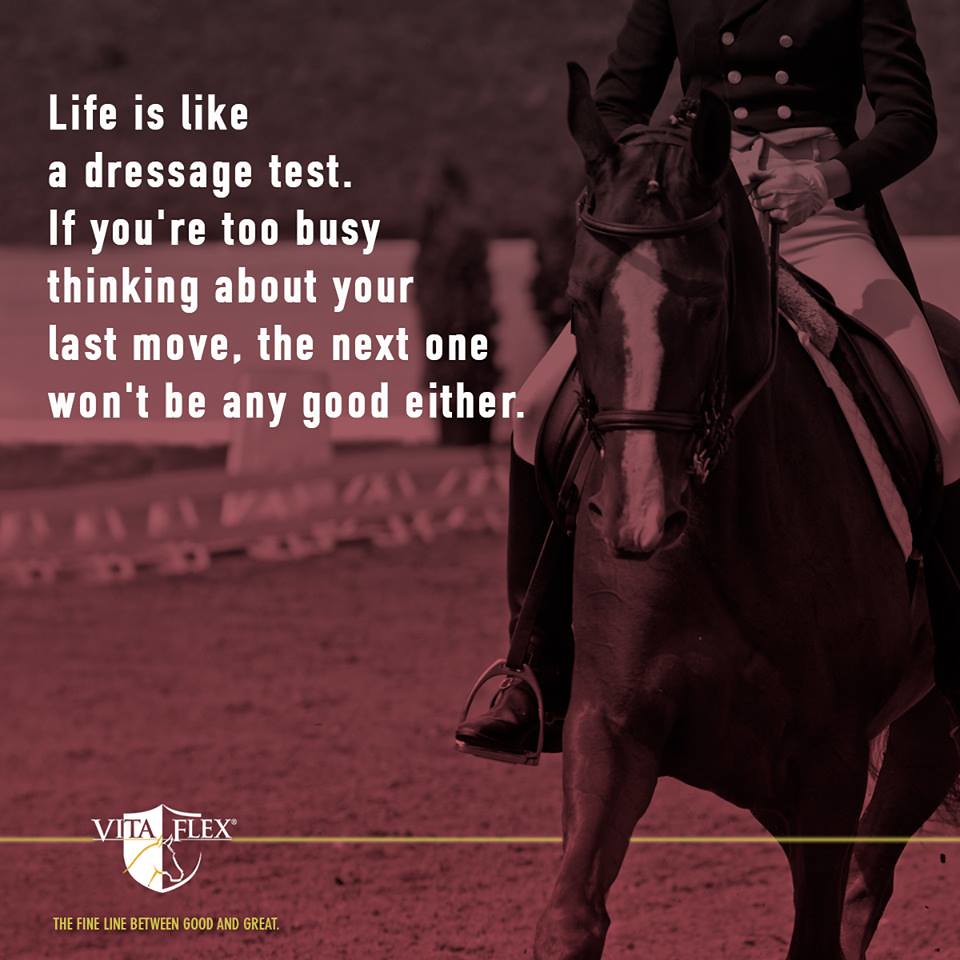This image, likely an advertisement for VitaFlex, features a rider atop a black-and-white horse in a sandy arena, reminiscent of a dressage setting. The rider, clad in a sophisticated equestrian outfit with a black jacket featuring six buttons, white pants, white gloves, and long black riding boots, holds the reins with precision. The horse, distinguished by a distinctive white strip running from its forehead to its nose, stands with one leg in front of and one behind a yellow line that seems ambiguously edited onto the photo. The text on the left side of the image reads, "Life is like a dressage test. If you are too busy thinking about your last move, the next one won't be any good either." At the bottom left corner, a VitaFlex logo—featuring a horse's head within a shield—accompanies the tagline, "The fine line between good and great." The entire image is overlaid with a heavy red tint, almost reducing it to a monochrome appearance.